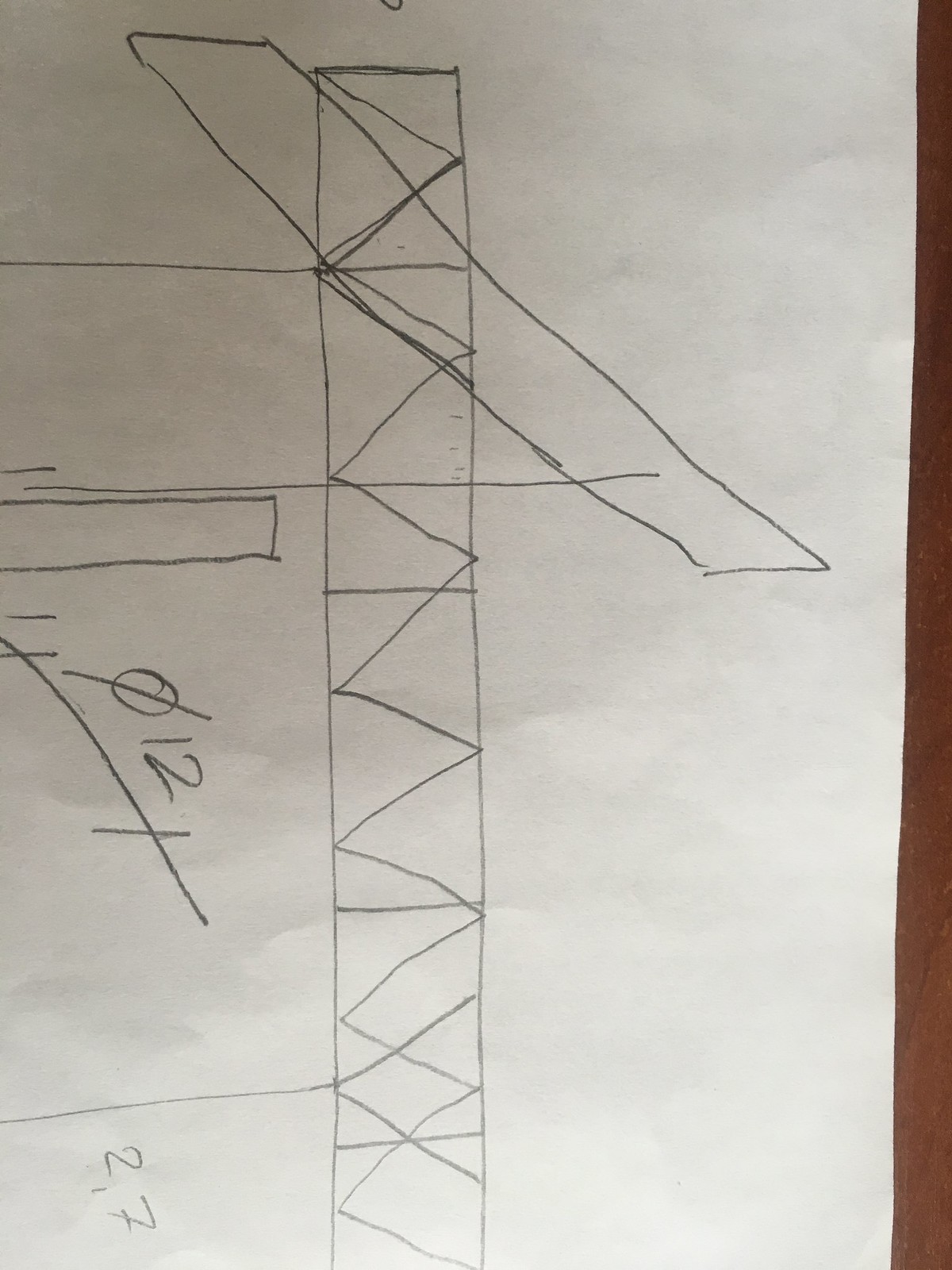The image depicts a white piece of paper with a prominent brown section on the right side, which transitions from dark brown at the top to a twilight brown at the bottom. Along the left-hand side, there is a symbol resembling a zero with a diagonal line through it. Running vertically from top to bottom is a stack of squares, arranged in a zigzag pattern. A diagonal line intersects the squares, extending from the top left to the bottom right of the paper.

To the left of the paper is a rectangle that stretches toward the center, reminiscent of a crane arm extending outwards. Below this rectangle appears to be a measurement marking of '27', accompanied by a line running from the left side to meet the end of the measurement.

The paper itself is not perfectly flat; it has slight wrinkles and ridges, along with some shading, giving it a textured appearance.